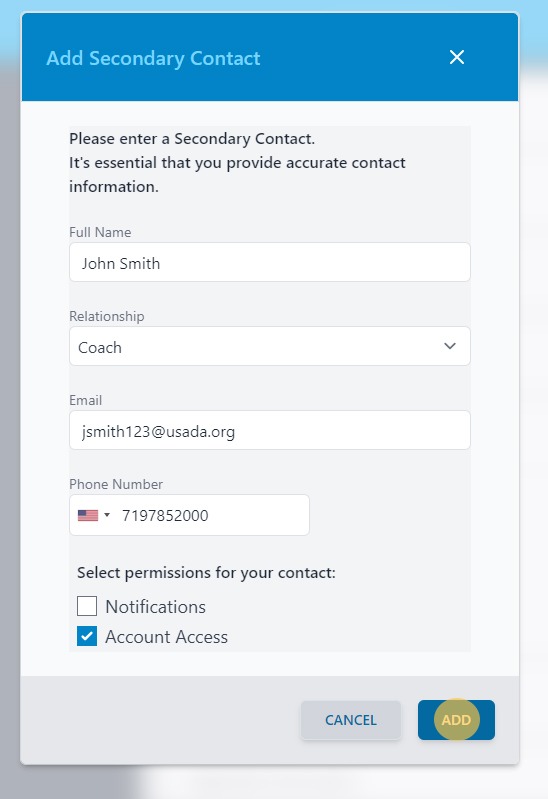A detailed screenshot capturing an interface from what appears to be a computer screen. Dominating the view is a large pop-up window which occupies approximately 97% to 98% of the screen's width and height. This window obscures a blurred background that transitions from light blue at the top, melding into a grey bar running vertically along the left-hand side, and then fading into white covering the remainder of the screen to the right.

The pop-up window features a blue header bar. On the left side of this bar, there is light blue text stating "Secondary Contact," and a white "X" icon on the right to close the window. The main body of the pop-up sports a very light grey background with black text prompting the user: "Please enter secondary contact. It is essential that you provide accurate contact information."

Below the prompt, there are several input fields filled out:
- **Full Name:** John Smith
- **Relationship:** Dropdown menu with "Coach" selected
- **Email:** jsmith123@usada.org
- **Phone Number:** An American flag icon followed by 719-785-2000

Further down, users are prompted to select permissions for the secondary contact. Two checkboxes are presented:
- **Notifications:** This box is unselected.
- **Account Access:** This box is selected and highlighted in blue.

Beneath these options is a slightly darker grey band featuring two buttons. On the left, a grey "Cancel" button with blue text. On the right, a blue "Add" button with a greenish-yellow circle and the word "Add" written in yellow at its center.

Overall, the screenshot clearly displays the details of the Secondary Contact pop-up window, including the necessary input fields and selectable permissions.